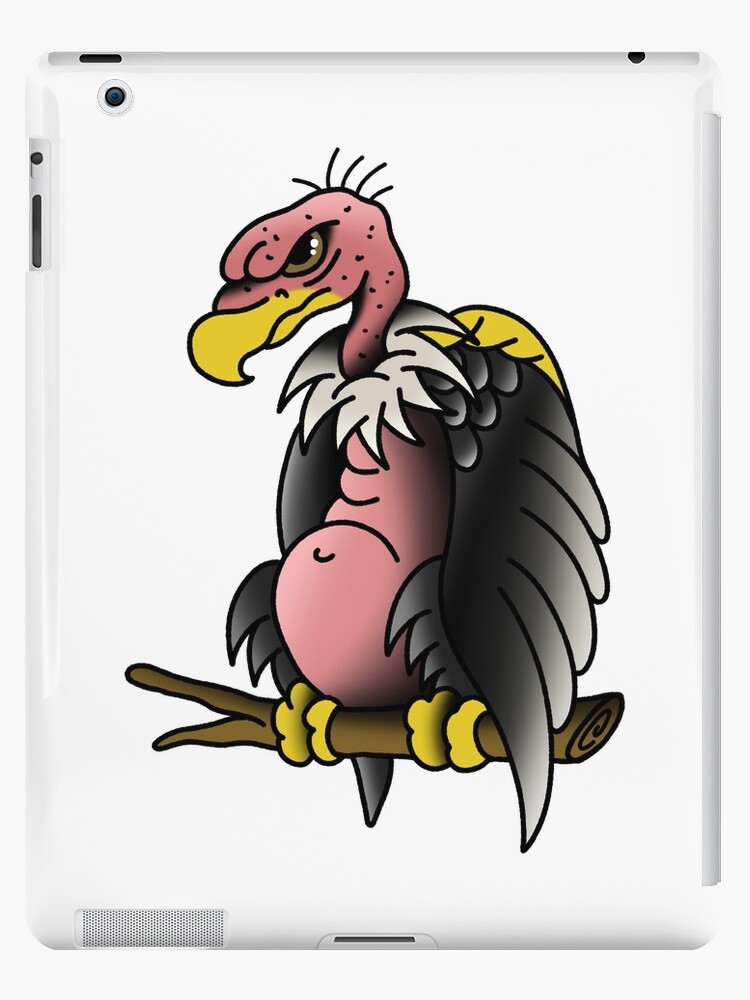The image features the back of a white tablet, possibly an iPad or laptop, with silver edges. Key elements include a camera on the upper right and charging ports at the top and bottom. Centered on the back is a high-quality, clear sticker of an animated cartoon vulture perched on a brown branch. The vulture has a distinctive appearance with a pink head, green eyes that appear very angry, a yellow beak, and numerous small black spots resembling warts. It sports five distinct tufts of hair on its head, white feathers around its neck, a red torso marked by lines suggesting a chubby belly, black wings, and yellow toes gripping the branch. The entire scene is set against a solid white background, brightly illuminated to highlight every detail. The image is devoid of any text or numbers, allowing the viewer to fully appreciate the vivid colors and intricate details of the vulture sticker.